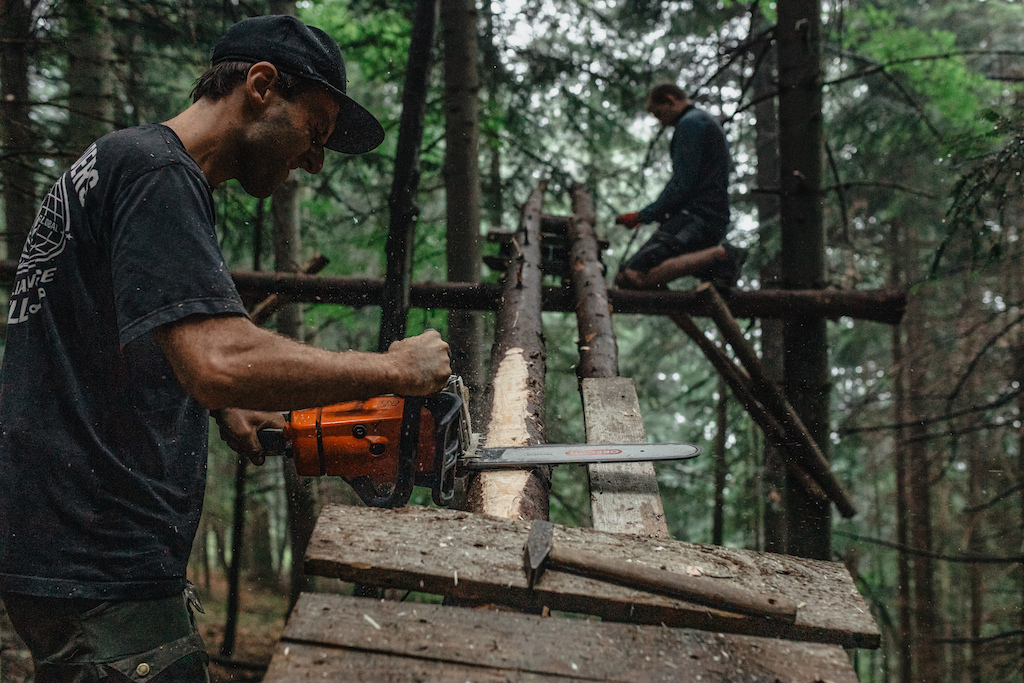In the midst of a dense forest, two white men, likely in their late 20s or early 30s, are engaged in woodworking, possibly building a shelter or cabin. The man in the foreground, sporting brown hair, a black baseball cap, a black t-shirt with an illegible white logo on the back, and black jeans, is intently shaving the bark off a large log with an orange chainsaw. His eyes are closed, perhaps in deep concentration. On the ground near him are a hammer, some wood planks, and two long parallel logs leading towards the second man.

The second man is elevated, kneeling on a log approximately 10-15 feet off the ground. He has blondish-brown hair and is dressed in a green long-sleeved shirt and shorts. He appears to be using his hands to work on the structure, possibly holding something orange. The backdrop is a vibrant mix of green leaves and dense foliage, with the forest floor covered in a carpet of brownish-orange leaves,, emphasizing the natural and rustic setting of their endeavor.